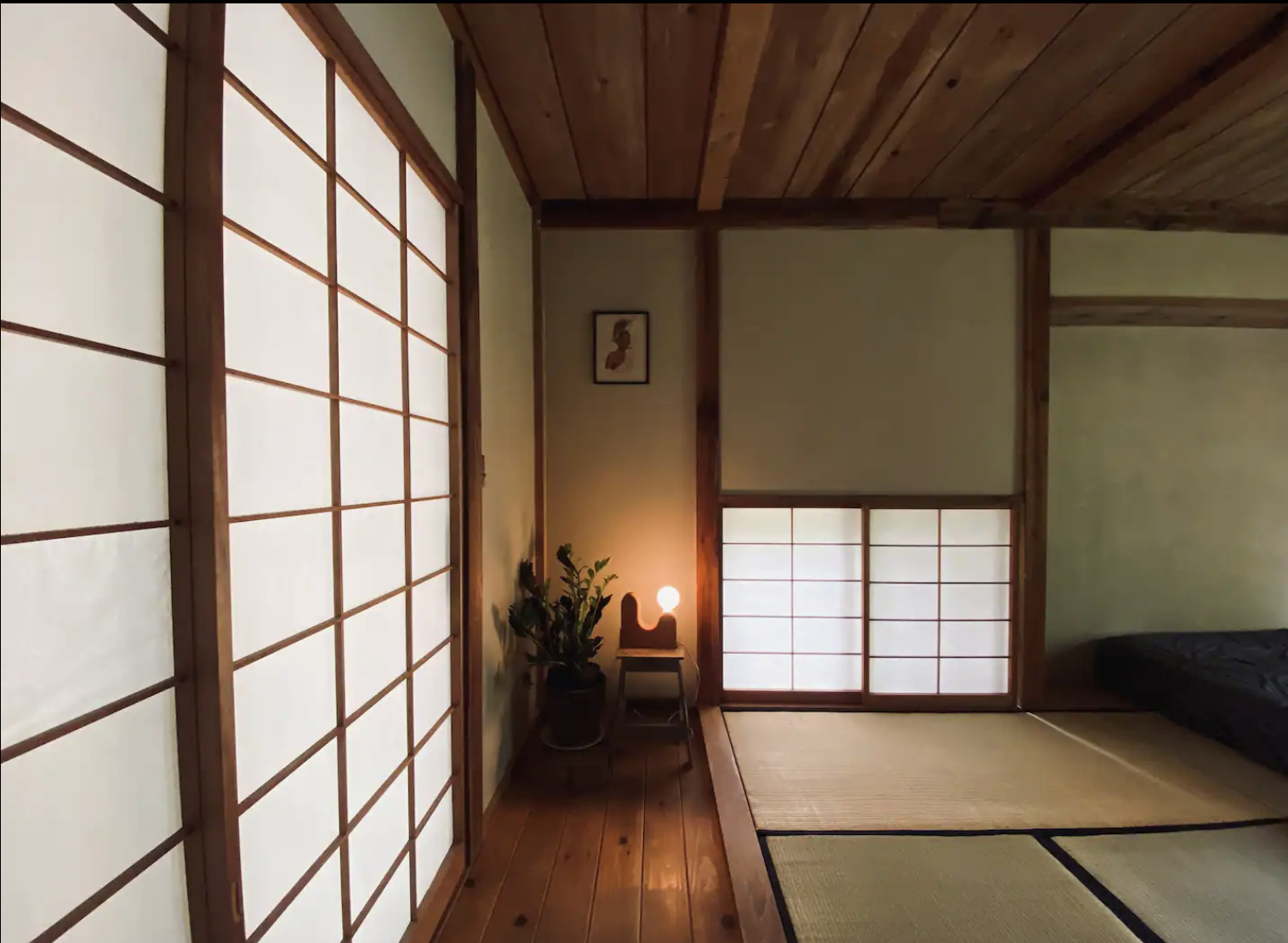The image depicts a traditional Japanese-style room characterized by sliding paper doors with bamboo and wood framing. The room features a wooden ceiling with visible grain and wooden bracing. The flooring consists of multiple tatami mats in green and tan hues, central to which lies a blue sleeping mat. The left wall is adorned with sliding doors, and wooden pillars accentuate the white and green walls. A small window above the tatami mats, also composed of wood and paper, complements the aesthetic. The room includes a single framed picture of a bird, hung in a black frame, with a ZZ plant in a pot below it and an adjacent small chair holding a light bulb. Despite some light in the room, it retains an overall dim ambiance, enhancing its serene, bedroom-like atmosphere.